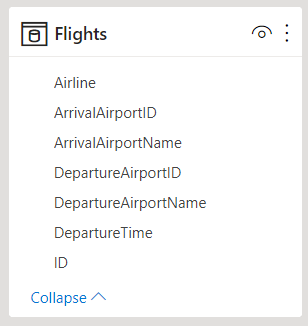A minimalist screenshot features a gray-bordered interface with a white background, likely from a phone or a larger web browser. Dominating the view is a small window labeled "Flights," accompanied by a simplistic icon—a plain rectangle with a smaller cylindrical shape inside—on its left. To the right of the "Flights" label are two icons: an eye symbol and an ellipsis (three dots).

Beneath the header, options are listed in a continuous string without spaces, suggesting a back-end setup rather than a consumer-facing application. The listed parameters include: airline, arrival airport ID, arrival airport name, departure airport ID, departure airport name, departure time and ID. 

Underneath these descriptions, blue text reading "collapse" features an upward-pointing arrow, indicating a clickable link. The overall design is stark, with black text and basic black icons, devoid of any images or decorative elements, reinforcing its utilitarian nature.